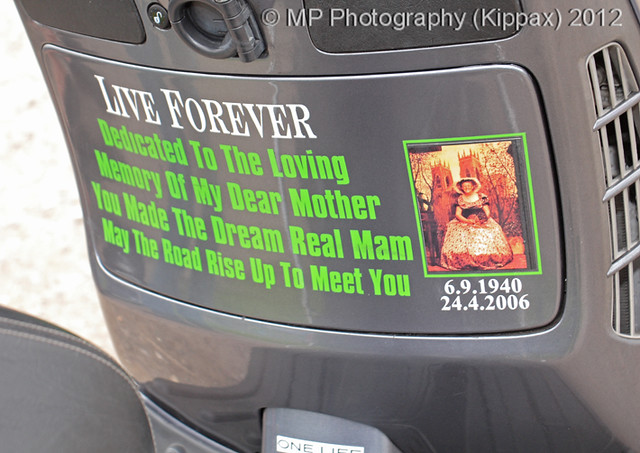This photograph features a dark gray, metallic object, possibly a rear console of a vehicle, displaying a detailed and personalized tribute sticker. Central to the image is a rectangular metal panel with curved edges, potentially a door or access panel, devoid of any handle. The object has a small button at the top center, portraying an unlock icon, suggesting an interactive or functional component.

In bold, uppercase white font across the center of this metal panel, the sticker reads "LIVE FOREVER." Beneath it, in a somewhat smaller, upper and lower case green font, it states, "Dedicated to the loving memory of my dear mother. You made the dream real, ma'am. May the road rise up to meet you." 

To the right of this heartfelt message is a square photograph in a light green border, depicting a seated woman. She dons a large, old-fashioned dress, potentially adorned with polka dots, and holds a fan in her right hand. Her attire, including a notable hat, evokes a medieval or historical aesthetic. The background of the photograph features what appears to be a castle with two spiked towers, adding to the vintage ambiance. The image has an orange tint, which gives it a nostalgic feel.

Below the photograph, white text marks significant dates: "6-9-1940" and "24-4-2006," indicating the birth and passing dates of the memorialized individual. At the bottom of the entire layout, where a license plate might usually reside, there's a gray panel with a small, white rectangle inscribed with "one life" in gray font.

The photograph captures both the beauty and intricacy of a personalized and touching memorial, combining elements of both past and present within a single, striking image.